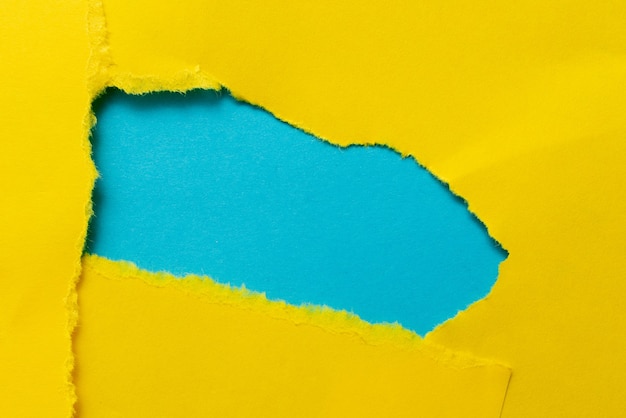The image depicts a detailed close-up of torn construction paper. The primary focus of the image is a jagged, uneven tear running across the middle of the paper. The top sheet is a bright yellow, with a piece torn away, revealing a light blue sheet underneath. The tear is irregular and starts slightly to the left, descending diagonally downwards to the right. There's an intriguing layering effect where parts of the torn yellow paper fold over and onto the blue paper beneath it, creating a sense of depth. Though some viewers suggest the top paper might include other colors like green or orange, the dominant visual elements are clearly the yellow foreground and the blue background. The photograph captures the textures and edges of the ripped construction paper, emphasizing the contrast between the vibrant yellow and the tranquil blue. The composition is wider than it is tall, adding to the visual impact of the tear and the contrasting colors.